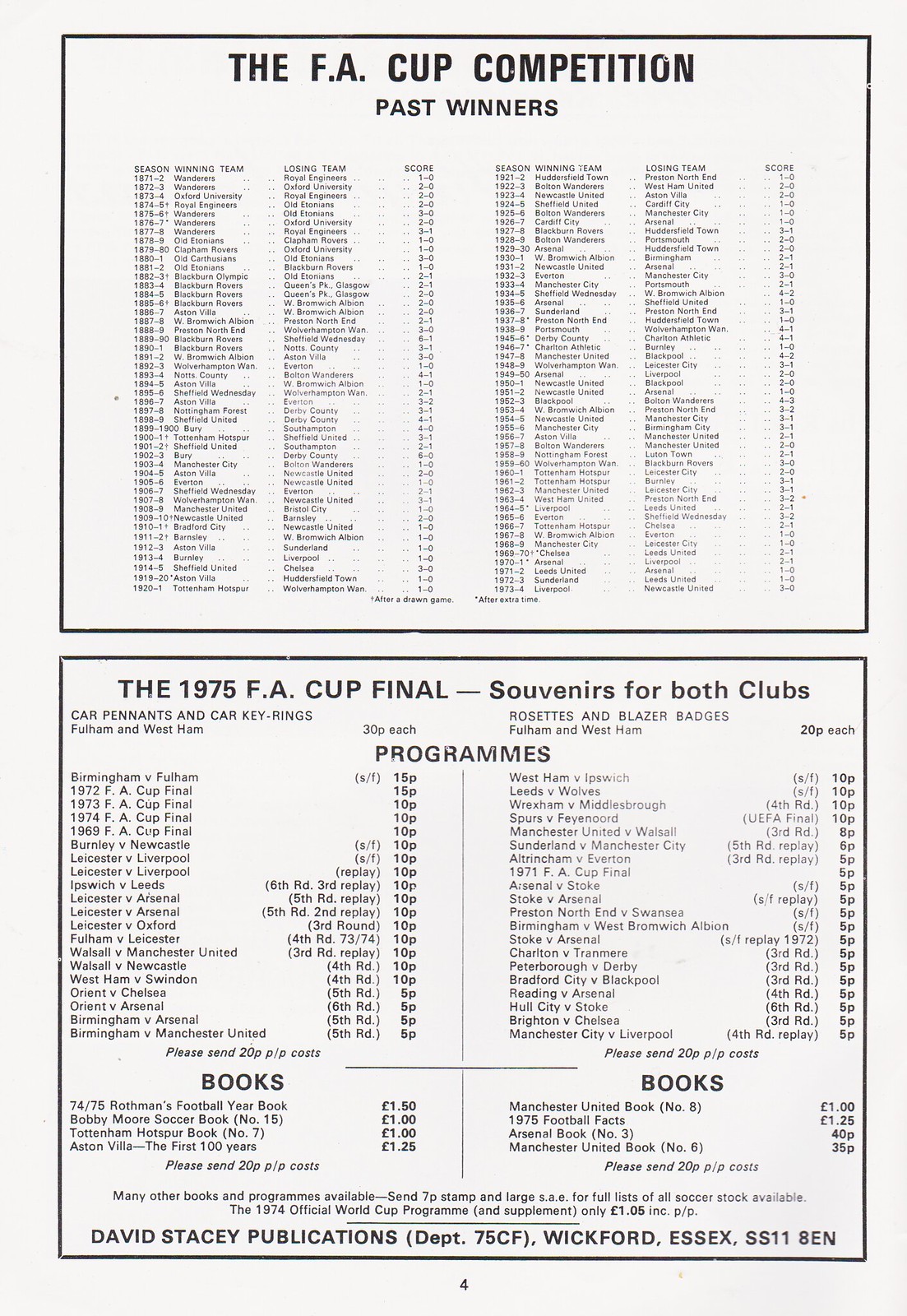The image depicts a black-and-white printed document featuring detailed information in two bordered sections on a white background. The top bordered area, outlined in black, is titled in bold capital letters "THE F.A. CUP COMPETITION - PAST WINNERS." Below this title, the section contains multiple columns of information, which appear to list the names of winning and losing teams, scores, and years, though the small print is difficult to read. The bottom bordered area also has a black outline and is entitled "THE 1975 F.A. CUP FINAL - SOUVENIRS FOR BOTH CLUBS." This section includes a variety of items labeled "programs" and "books" with corresponding prices. Items listed include programs priced at 10p, 15p, or 5p, and books such as the "74/75 Rothmans Football Yearbook" for £1.50 and "Manchester United Book No.8" for £1. At the very bottom of the document, it reads "David Stacey Publications, Department 75CF, Wickford, Essex, SS118EN."